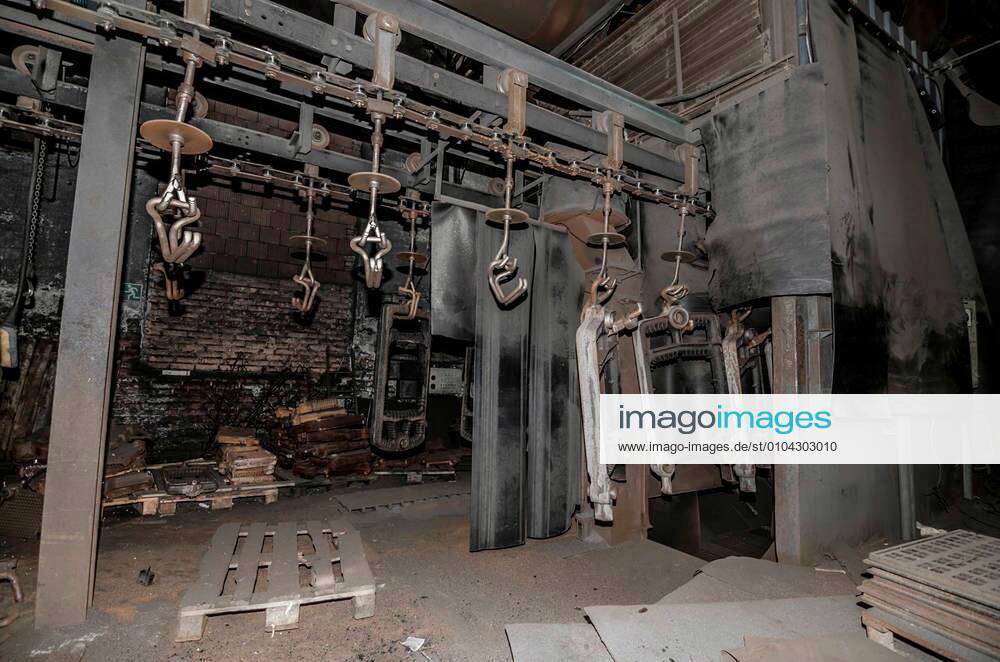The photograph captures the interior of a worn and cluttered workshop or industrial site. Dominating the scene is a gray cement floor, dirty and dust-laden, strewn with a few wooden pallets. Against the backdrop of an aged brick wall, metal racks stand mid-ground, from which hang several silver metal hooks, empty and gleaming. To the right side of the image is a designated storage area, containing various sharp tools and other materials. Over the image, a banner reading "Imajo Images" in black and blue text is visible, including a URL and a specific ID number, lending an organized yet gritty atmosphere to the workshop space.